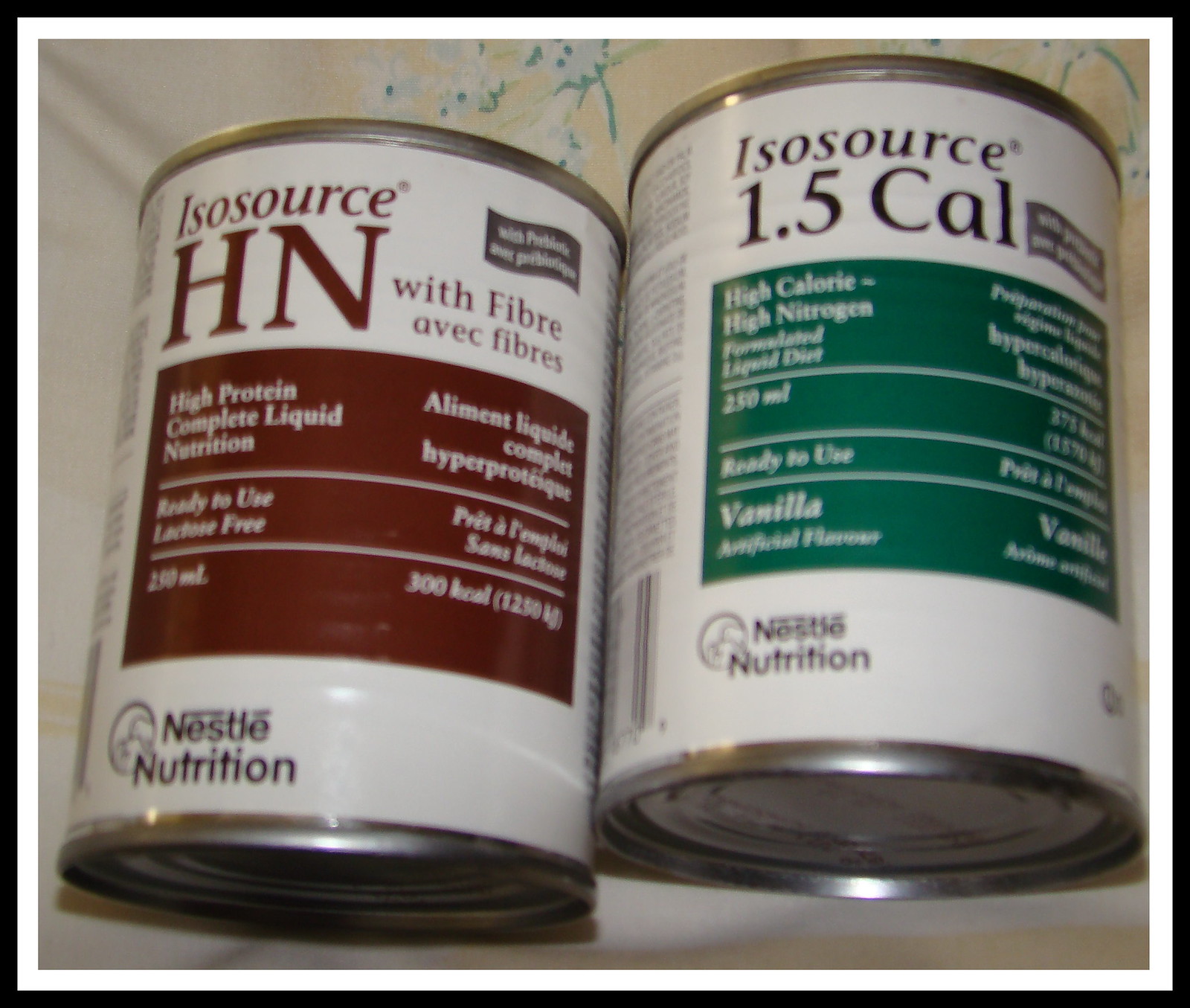This close-up color photograph captures two cans of nutritional liquid supplements lying on their sides on a yellow floral fabric background. The can on the left features a white body adorned with a dark red label. The label reads "Isosource HN with Fiber" and lists several details including "AVEC fibrous with probiotics and prebiotics," "high protein complete liquid nutrition," "aliment liquid complete hyperproteic," "ready-to-use lactose-free," and "PRIT, a lympha sans lactose." The can has a volume of "290 milliliters (300 equal to approximately 1250 kilograms)." The bottom of the label bears the "Nestlé Nutrition" logo.

The can on the right is similar in design but distinguishes itself with a green label. This label states "Isosource 1.5 Cal" and highlights it as a "high calorie, high nitrogen formulated liquid diet." It also notes the content as "250 milliliters" with a "ready-to-use vanilla artificial flavor." There are additional words on the right side of the label in another language, which appear out of focus. The label on this can also concludes with the "Nestlé Nutrition" insignia. The vibrant yellow fabric with floral patterns underneath adds a touch of warmth and texture to the scene.